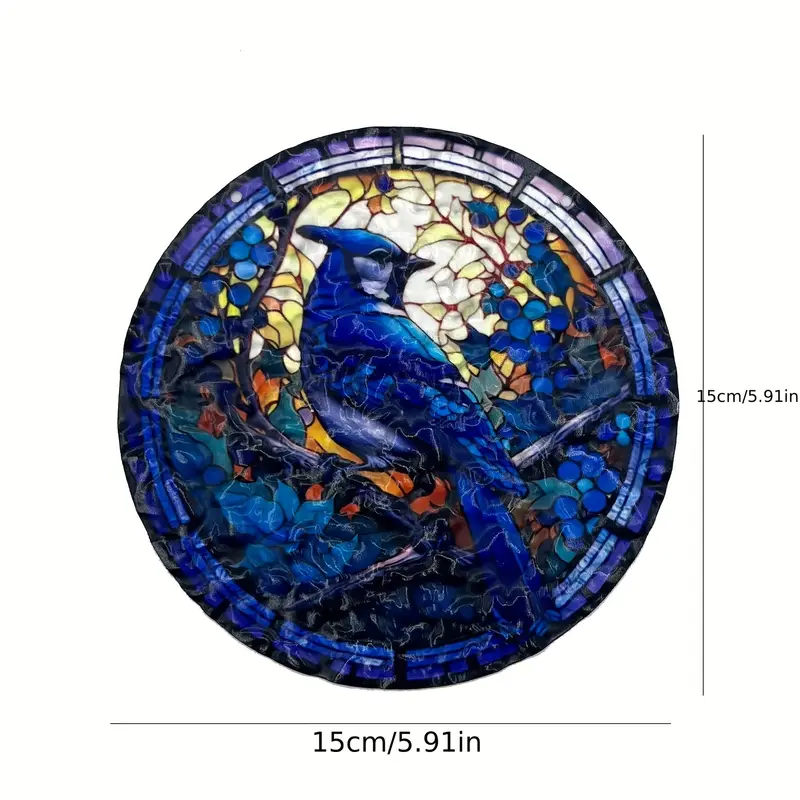This is a color photograph of a round stained glass suncatcher, measuring 15 centimeters (5.91 inches) in diameter as indicated by the measurement lines on both the right side and bottom of the image. The central focus of the stained glass is a blue jay bird, depicted in royal blue and varying shades of blue. The bird is perched on tree branches, with its body facing left and its head turned to the right, showing a side profile with distinctive features such as a peaked head, black eyes, and a black beak. The background behind the bird is composed of stained glass fragments in vibrant yellow, orange, and white colors. Surrounding the bird are images of flowers and additional branches, primarily in shades of blue, accented with orange and yellow leaves. The entire scene is set against a pure white background, making the intricate details and colors of the stained glass artwork stand out prominently.